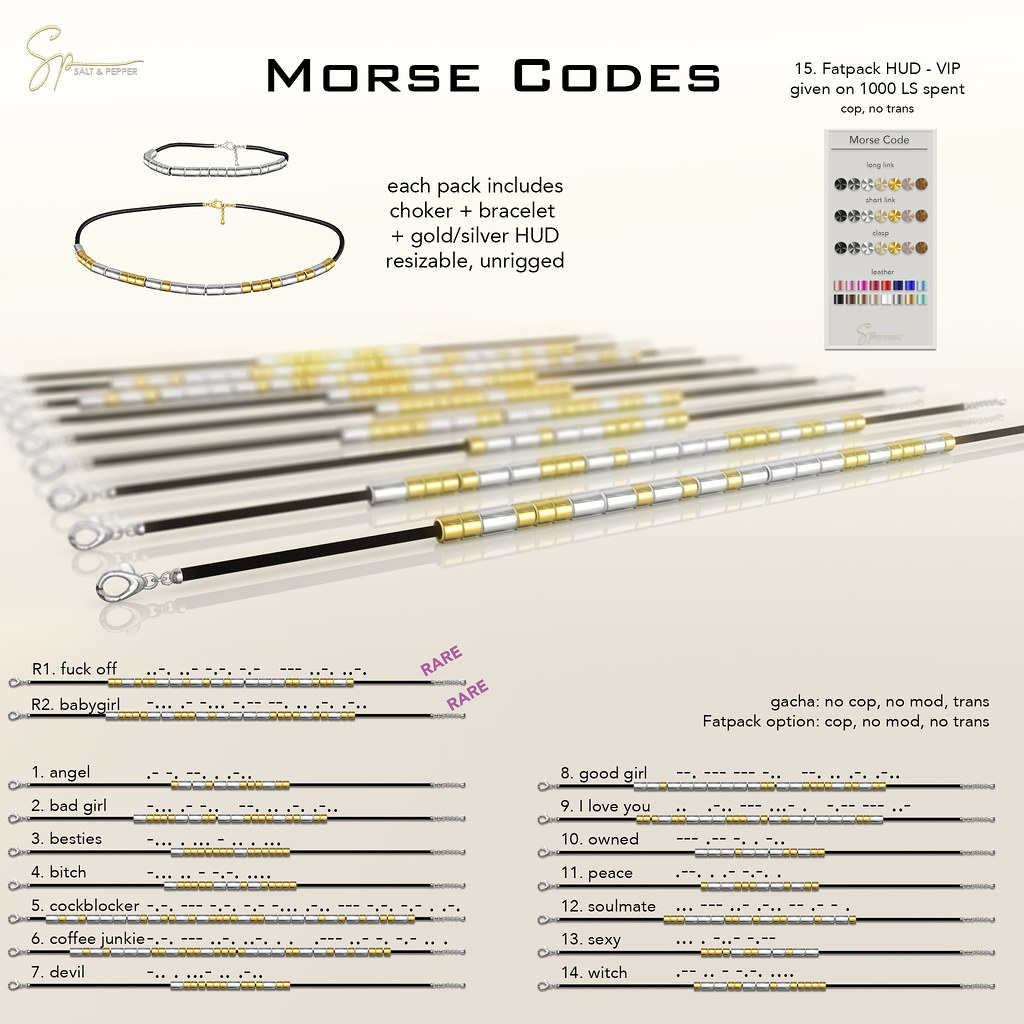The image showcases a collection of distinctive jewelry comprising a choker and a bracelet against a white background. Prominently at the top, bold black letters spell "Morse Codes." Each jewelry pack includes both a choker and a bracelet, accompanied by a HUD for gold and silver customization, and is described as resizable and unrigged. The jewelry pieces are laid out in a neat line, featuring gold and silver beads arranged in patterns resembling Morse code, representing various words and phrases. Some phrases are playful or inspiring, such as "angel," "bad girl," "coffee junkie," "sexy," "witch," "peace," "I love you," and "good girl," while others include more profane language like "F off." The image also contains a small chart depicting different colored dots related to Morse code, a view of a silver clasp on a black thread, and details like a ring and hook clasp mechanism for secure fastening.